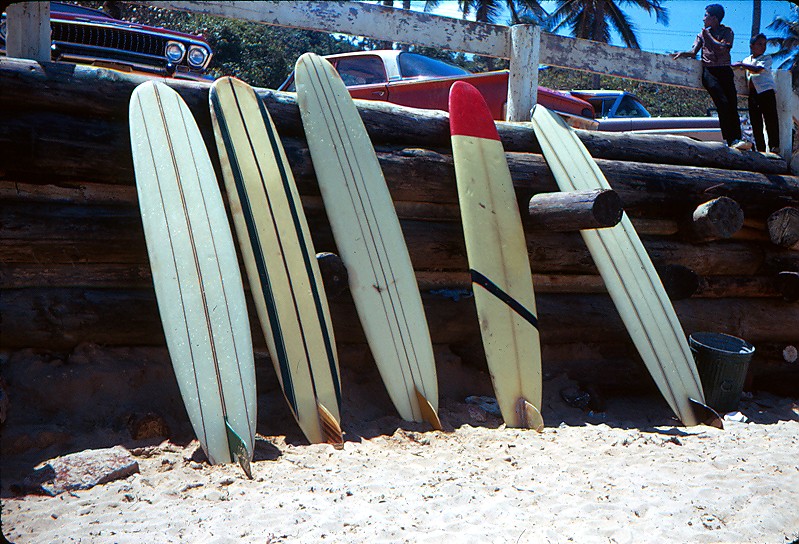The photograph captures a picturesque beach scene with a row of five weathered, older surfboards propped up against a dark brown wooden log wall, which acts as a barrier between the sandy beach and an elevated parking lot. The beach sand transitions from light tan to white, and there's a scattering of rocks towards the water's edge. Each surfboard has unique distinguishing marks: an off-white one with a brown stripe, a yellow board with dark blue striping, another off-white with brown accents, a yellow one featuring a black diagonal stripe and a red tip, and a final off-white board with brown striping. The surfboards bear the marks of time, indicated by their banged-up and distressed appearance. Above the log wall, the parking lot hosts three vintage cars, including a red and white vehicle. Two African-American children stand on the ledge between the log barrier and the parking lot. The background features palm trees that frame the bright, blue sky, enhancing the quintessential California beach town vibe. A metal bucket, possibly a trash can, is positioned next to the last surfboard, casting a shadow over the sandy beach.